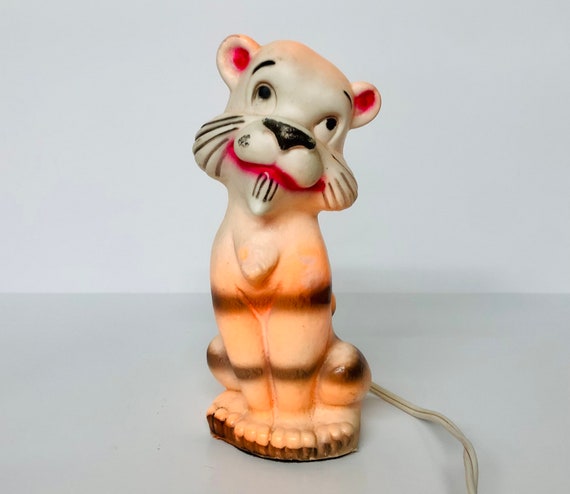The image depicts a small, cartoonish tiger lamp, ideal for a child's room, characterized by a power cord extending from the back of its base. The tiger is in a sitting position with all four paws aligned forward and its rear hunched similarly to a circus tiger on a drum. It has a slightly cocked head, looking lovingly up to its left. The tiger is predominantly orange with darker brown stripes around its chest and leg area. Its face features black painted whiskers, a black nose, and expressive eyes gazing upwards with a smile. Notable details include pink inner ears, a white face, a reddish mouth, and a dark brown base. The lamp illuminates from the shoulder blades down, leaving the head unlit, and is set against a white background.